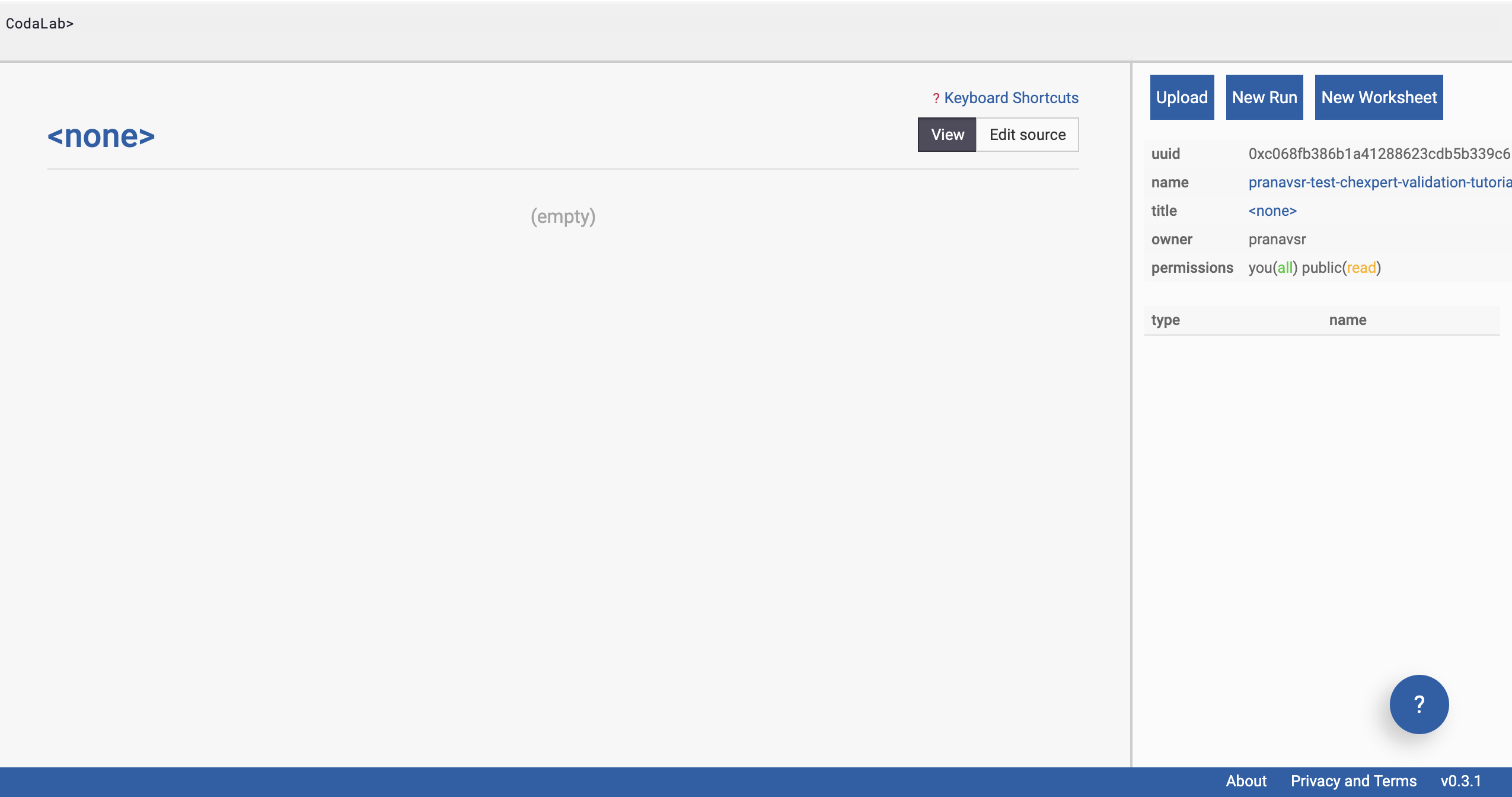This image showcases a screen from a coding program, likely part of a development environment called "Codelab." The screen is oriented in landscape mode and predominantly features shades of gray with some blue elements.

At the top of the screen, a long rectangular gray box stretches across, delineated by a thin gray line. Within the upper left-hand corner of this box, the black text reads "Codelab," with a right-pointing arrow adjacent to the "D" in "Codelab." This signifies the start of the navigation or hierarchy within the program.

Beneath this top section, occupying approximately 75% of the screen's length, is another gray box with a subtle border at the top. Breaking up the rectangular space within this gray background is a small box at its top section. To the bottom left of this small box, the word "None" is displayed, flanked on either side by carets (< and >).

To the right of the "None" label is a black box labeled "View," which contrasts with an internal white section. Adjacent to this box is an "Edit Source" button. Following this, a red check mark appears next to text that reads "Keyword Shortcuts," highlighted in blue. Directly beneath this, another box labeled "Empty" can be observed.

On the far right of the screen is a vertical white box featuring blue buttons with white text labeled "Upload," "New Run," and "New Worksheet." 

Further below, the screen displays several coding options, presented in a list format. Categories such as "UUID," "Name," "Title," "Owner," and "Permissions" are listed, each with corresponding detailed information that is likely pertinent to various aspects of coding or project management.

At the very bottom right of the screen, a blue circle contains a white question mark, presumably a help or information icon for user assistance.